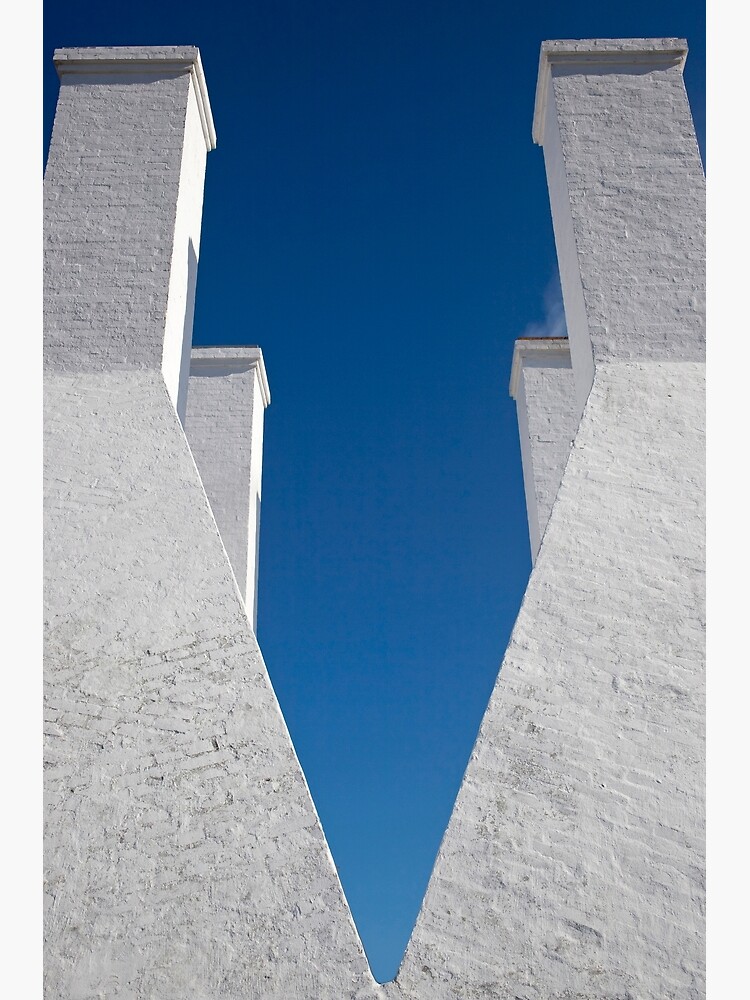The vertically aligned rectangular picture captures a striking architectural scene against a crystal-clear blue sky. Dominating the image are two towering stone columns that create a V-shape as they taper inward toward each other. These columns, composed of white or light gray bricks, feature square, flat tops and vertical rectangular sections that broaden at the base. On closer inspection, the structures resemble massive chimney stacks, with four of them arranged in a triangle-shaped pattern. From the rightmost chimney, wisps of white smoke hint at activity within the building. A tiny cloud, which might actually be smoke, adds a subtle disturbance to the otherwise pristine sky. The photograph appears to be taken from the roof, looking upwards, emphasizing the grandeur of the chimneys and the vivid blue expanse above.